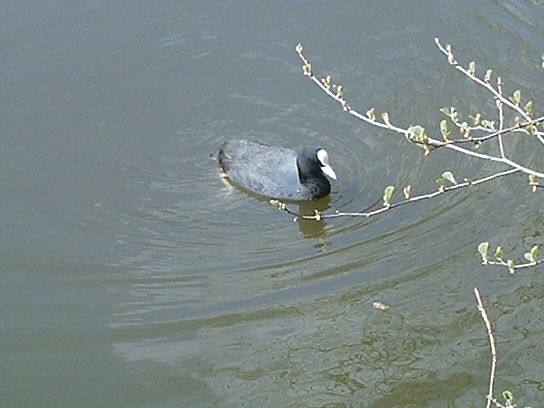This outdoor photograph features a duck centrally positioned in a body of water, possibly a pond or lake. The water, a greenish-brown hue, is gently rippling around the duck as it travels towards the right. The duck has distinctive coloring: a white bill and forehead, a charcoal-colored head extending into the front of its body, and a dusky gray body. You can see the duck's yellowish-orange feet beneath the water's surface. Thin tree branches with tiny green buds and leaves extend from the right side and lower right corner of the image, suggesting early spring. Despite being a bright day, the sunlight appears diffused, casting a subtle shimmer on the water. There's no visible shoreline, giving the impression of an intimate, tranquil scene.